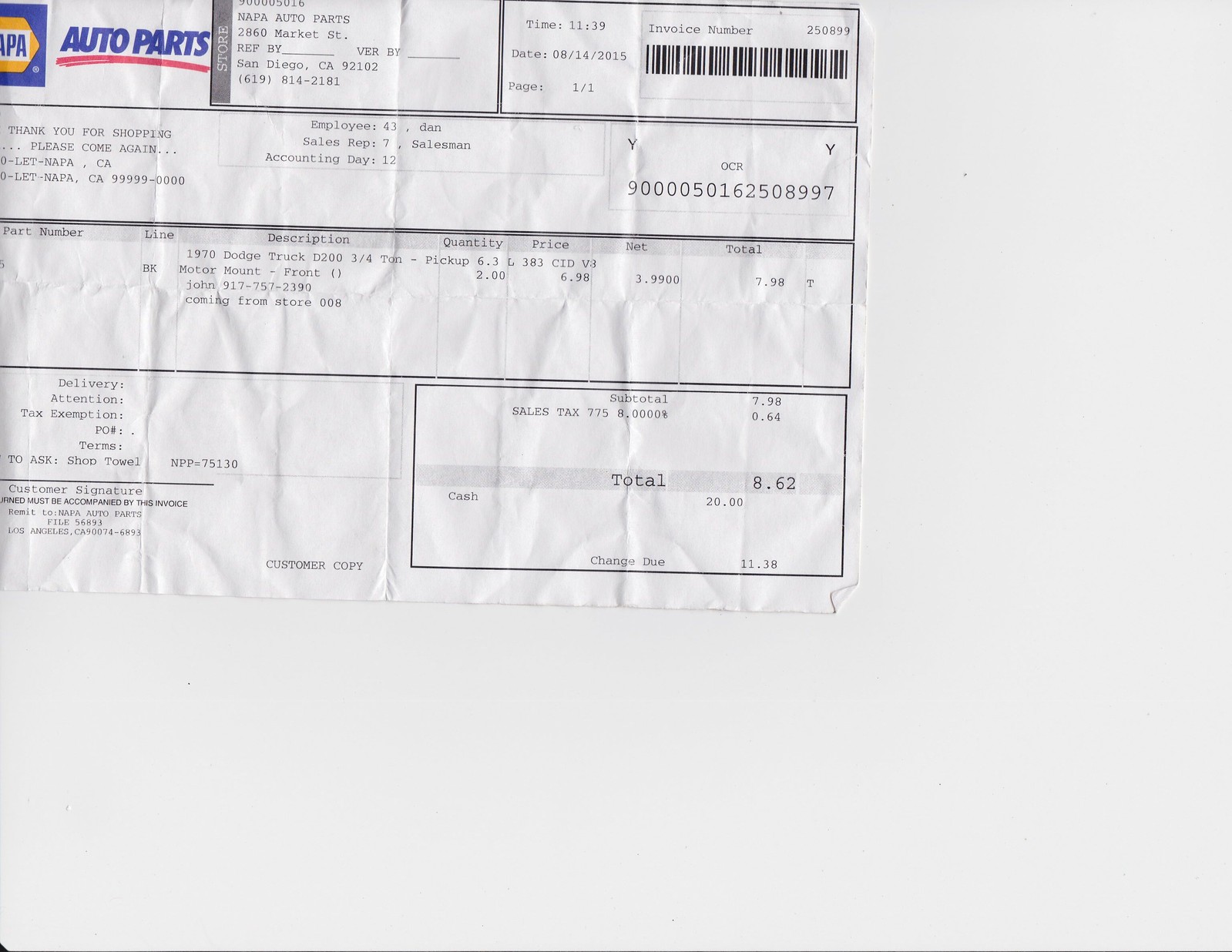Detailed Caption: 

"This is a detailed shopping receipt from NAPA Auto Parts, located at 2860 Market Street, San Diego, California. The receipt, printed in black and white, indicates a total amount of $8.62 for various auto parts. The transaction was handled by Sales Representative Dan, and the accounting date was the 12th. The customer paid in cash and received this customer's copy that includes specifics like the order number, invoice number, and a note indicating it was tax-exempt delivery. The receipt also features NAPA Auto Parts' iconic logo, which is designed in blue with a red line, and their name, displayed in bold yellow and blue."